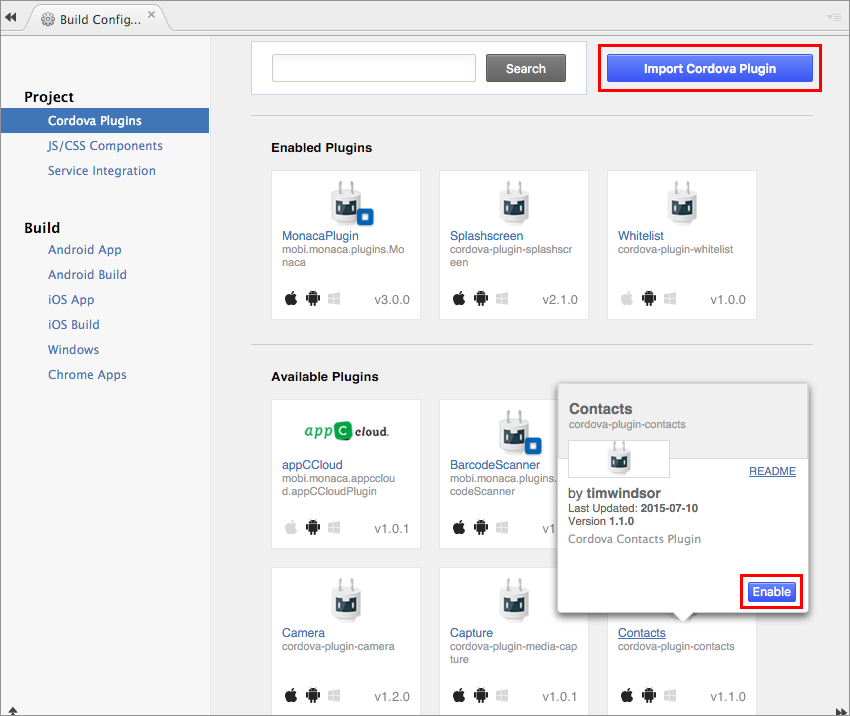**Detailed Caption:**

The screenshot captures a detailed view of a software build application, specifically related to Cordova plugins. The interface is predominantly pale blue, creating a clean and subtle background. On the left side of the page, a vertical column enumerates various selections in a segmented, tab-like display. At the top of this column, "Build Config" is presented as a file-folder-style tab.

The column's header, "Project," is highlighted in black text, followed by a series of blue-highlighted options with white text: "Cordova Plugins" is currently selected. Beneath this, the options "JS / CSS Components," "Service Integration," and a "Build" section appear in smaller print, with subsections like "Android App," "Android Build," "iOS App," "iOS Build," "Windows," and "Chrome Apps."

To the right of this column and spanning the majority of the page is a workspace with a continuous pale blue background. At the top of this workspace, a centered text search box set against a white backdrop allows for quick plugin search, while to its right, a prominent blue "Import Cordova Plugin" button with a distinctive red border is visible.

Below this section, the interface is divided to display "Enabled Plugins." Here, three plugins ("Monica Plugin," "Splash Screen," and "Whitelist") are shown with small plug icons. A thin, probably black or dark blue line demarcates this from the "Available Plugins" area below, which lists plugins like "App," "C Cloud," "Barcode Scanner," "Camera," "Capture," and "Contacts" in a structured grid format of two rows containing three plugins each.

A small pop-up window overlays the "Contacts" plugin, providing specific information about the "Cordova Plugin Contacts" by Tim Windsor. Details such as the last update date (2015-07-10) and version are noted, with a clickable blue "Enable" button bordered in red positioned in the bottom right corner of the pop-up.

Overall, the interface appears user-friendly and is systematically organized to enable efficient navigation and clear overview of available and enabled plugins.